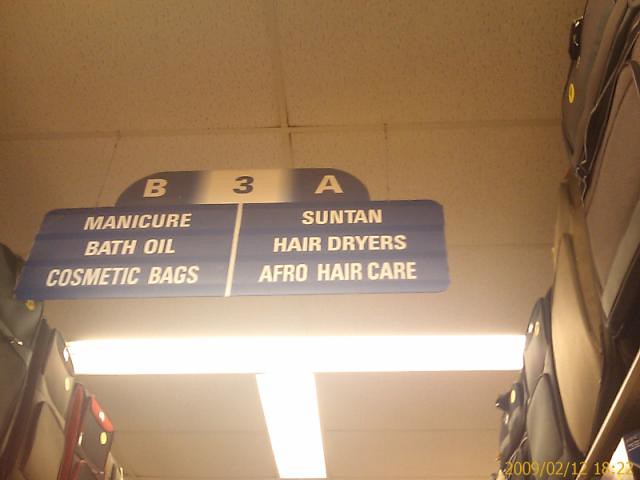This image captures an indoor scene from a store, taken from a low angle looking upward, possibly by someone standing below. The photograph's perspective emphasizes the detailed, standard white rectangular ceiling tiles, each bordered by thin gray lines and speckled with minuscule dots. The ceiling also features slim, rectangular lights that softly illuminate the store interior. An additional element suggesting the view might be from a security camera is a timestamp displayed in yellow text at the bottom right corner, reading "2009/02/12 18:22."

Hanging prominently from the ceiling is a blue sign with white text, divided into two sections: one side reads "B3A ILB," listing "Manicure, Bath Oil, Cosmetic Bags," while the other side marked "A" advertises "Suntan, Hair Dryers, Afro Hair Care." Below this sign, the top shelves are lined with an array of suitcases, stacked in neat rows, providing a stark contrast to the clean and orderly ceiling above.